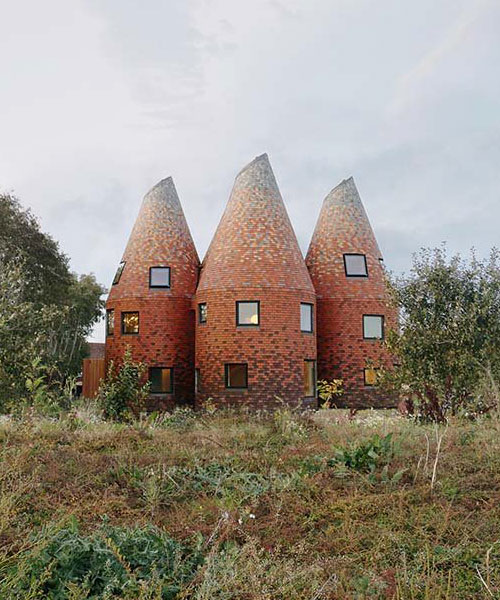The image depicts an outdoor scene under a mostly cloudy sky with patches of blue. In the foreground, the left side features a taller tree with some bushes in front, while the right side showcases smaller trees with slender trunks, surrounded by grassy areas, small brush, and weeds. The focus of the image is on three unique, red-brick buildings positioned in a near triangular arrangement. These round structures rise to truncated conical tops, resembling the slanted tip of a crayon. Each building has an array of square and rectangular windows that are irregularly placed across three floors. The setting creates a somewhat whimsical contrast with the rustic yard of scraggly grass, bushes, and brambles, all under a gray, overcast sky.